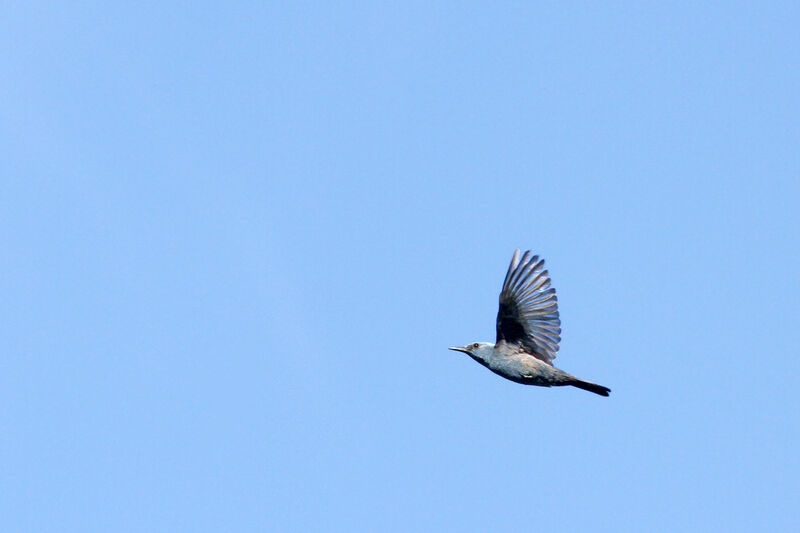This color photograph, captured in a landscape orientation, provides a majestic view looking up at a bird in mid-flight. The bird, seen in profile, soars from the right to the left side of the image. It is a small to medium-sized bird, characterized by its light gray plumage, long pointed beak, and dark tail feathers. The bird has its wings fully extended upward in a vertical position, with the feathers fanned out, creating a graceful arc to the right. This dynamic pose is set against a serene, light blue sky that fills the entire background, enhancing the bird's form. Positioned about a third of the way up the height of the image, the bird is the focal point of this beautifully detailed and realistic photograph, likely taken using a drone or from an elevated vantage point.